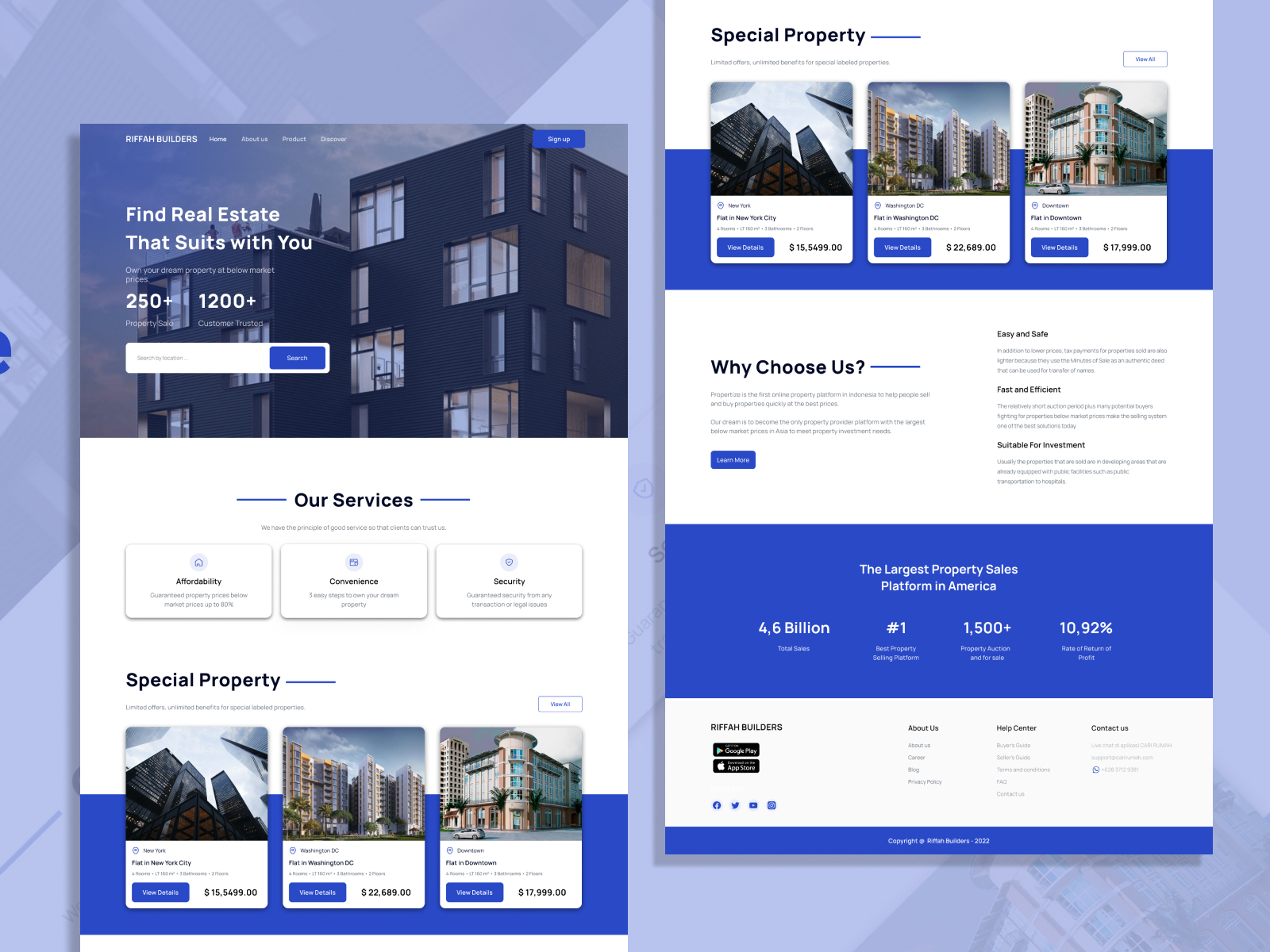### Descriptive Caption for Image of Real Estate Webpage

The screenshot captures a webpage dedicated to real estate services. The overall background of the webpage is a soothing cobalt blue, overlaid with stylized images of city streets and buildings, evoking an urban landscape theme.

On the left side of the webpage, there's a distinct vertical section featuring a prominent photograph at the top. This image showcases a sleek, modern apartment or high-rise building. Superimposed on this photograph in clean, white text is the phrase "Find real estate that suits you." Below this text, numeric values "250+" and "1,200+" are displayed, possibly indicating the number of participants and properties listed, though this is not explicitly clarified. A search bar with a blue-buttoned search function is positioned underneath these numbers. Further down, the section is titled "Our Services," featuring three horizontally aligned rectangles that likely serve as menu options, although the labels are illegible.

The lower portion of the left section is dedicated to "Special Property," presenting three featured properties. The first property image on the left displays a sleek glass high-rise, the middle showcases a more traditional high-rise building, while the third image on the right highlights a uniquely modern structure with a rounded design.

The right side of the main image mirrors the left side with another vertical page. At the top, this page is labeled "Special Property" and features the same three images found at the bottom of the left page, complete with listed prices and actionable buttons. This creates a cohesive continuation between the two sections.

Beneath these images, a white rectangle occupies the middle third of the right page, containing a section titled "Why Choose Us," accompanied by detailed fine print text and a button presumably linked to more information.

The bottom portion returns to a cobalt blue background, featuring a bold statement: "The largest property sales platform in America." The section also includes various statistics such as "4.6 billion," "number one," "1,500+," and "10.9 percent," though the significance of these numbers is undisclosed due to their tiny labels.

The design is modern and user-friendly, oriented towards individuals seeking detailed and accessible real estate information.